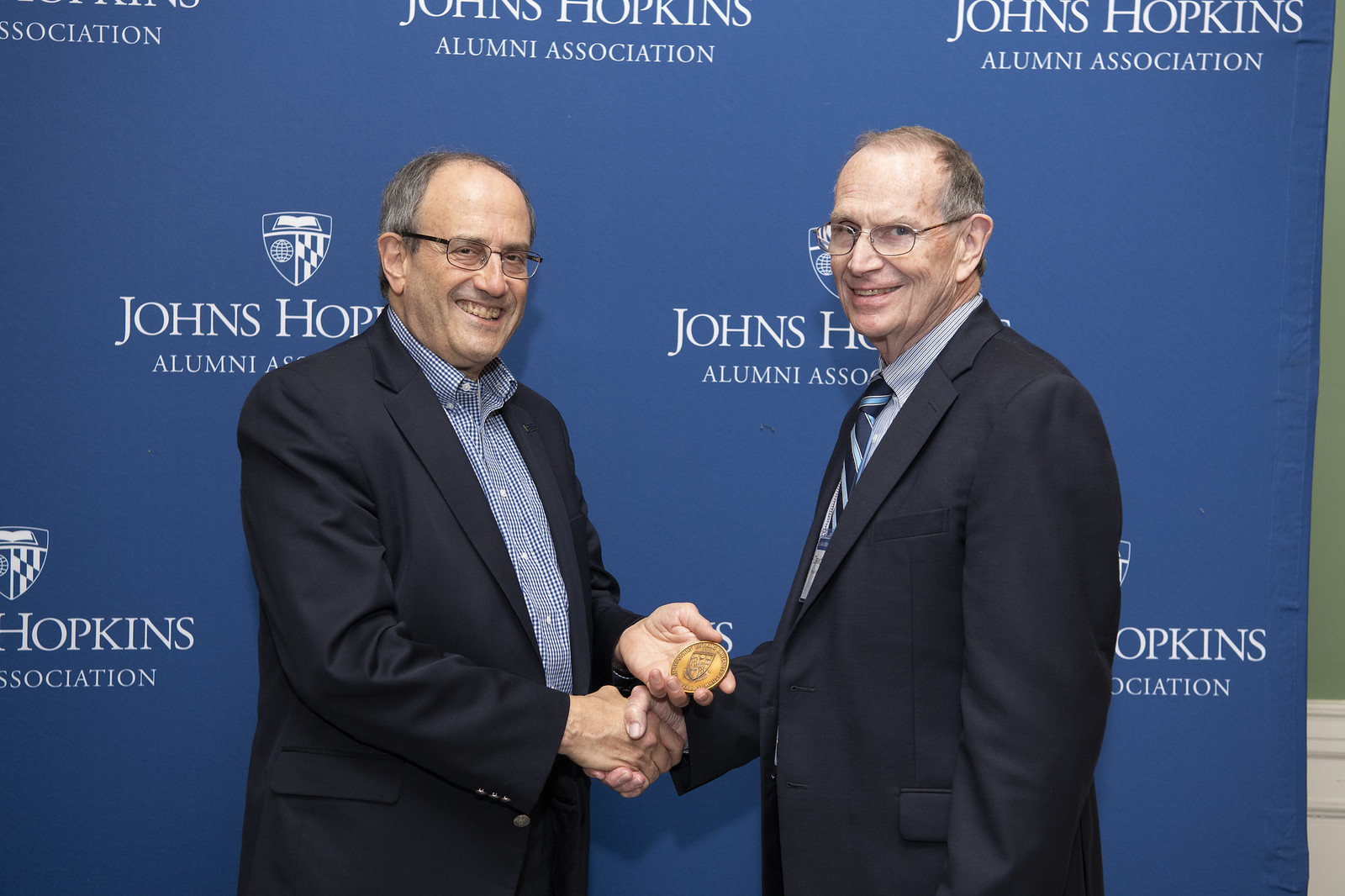The image showcases two elderly men standing in front of a backdrop emblazoned with the words "John Hopkins Alumni Association" in white lettering over a blue background. Both men are dressed in black suit jackets, though their attire underneath differs slightly. The man on the left, who has balding gray hair and wears black rectangular glasses, is smiling broadly. He is clad in a checked blue and white shirt without a tie and is shaking hands with the man on the right. In his other hand, he holds a gold-colored medal featuring the John Hopkins emblem. 

The man on the right, slightly balding with light brown hair and gold-framed oval glasses, sports a light blue and dark blue striped tie. He, too, is smiling, though his smile is more subdued. The two men appear to be participating in some form of award ceremony, likely recognizing contributions or achievements within the John Hopkins Alumni Association, with one man presenting a medal to the other.